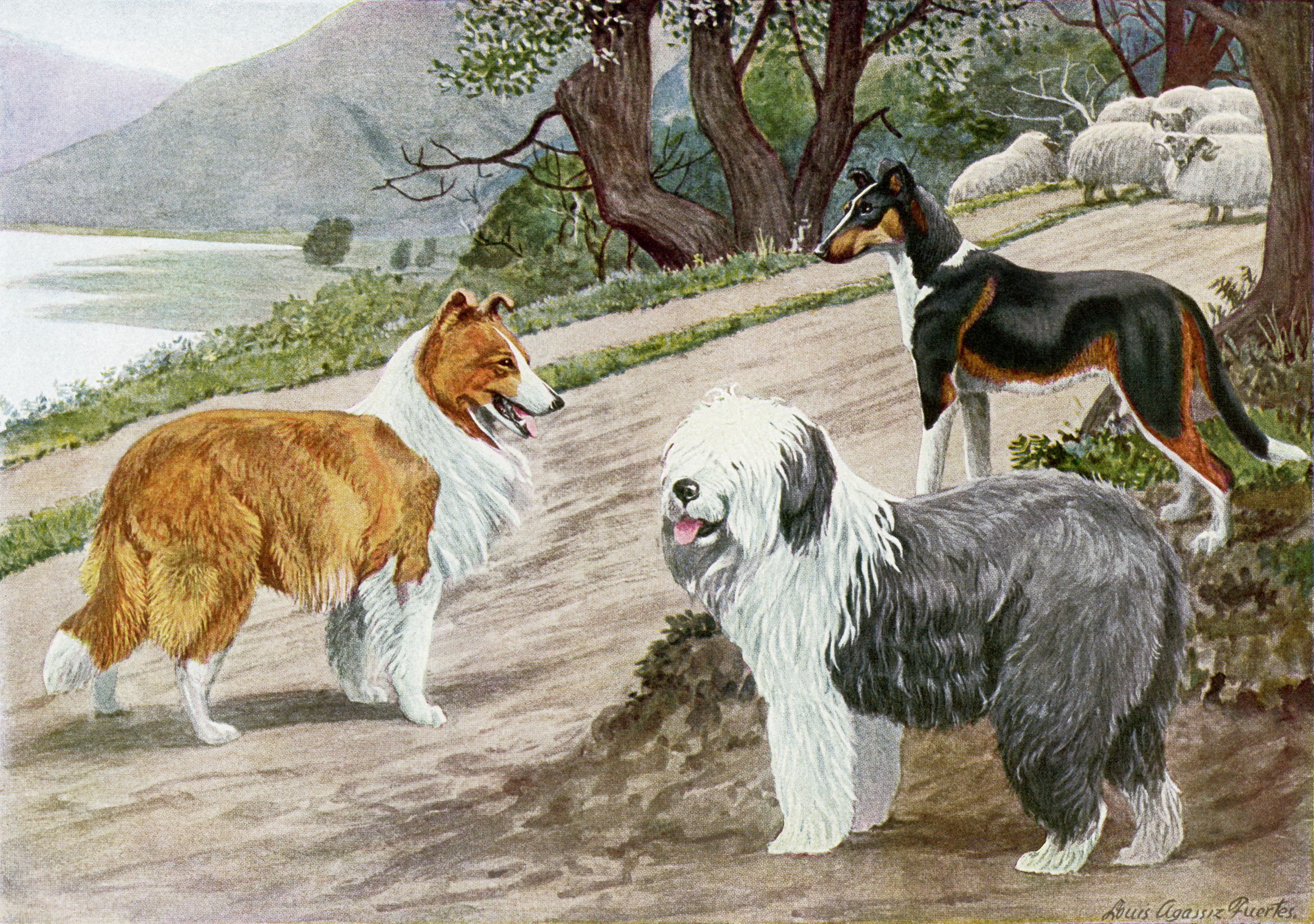This is a detailed and professionally done drawing of three dogs placed in an outdoor setting featuring a lake, trees, and mountains in the background. The artwork, likely created by Luis Agassi Fuentes, portrays the dogs standing on a dirt path with fluffy white sheep in the distance. The poster is wider than it is tall, showing a border collie with a distinctive brown and white coat, looking alert with perky ears. To its right stands an old English sheepdog with a grey body and a mane of white fur, including white legs and small white paws. Above these dogs on the path, there is another dog possibly resembling a tricolor smooth-haired collie, with a black top and brown underbelly fading to white on the lower legs and belly, and featuring a slender nose and slightly bent ears. The serene composition also includes a central lake, mountains lightly shaded with charcoal, and a road intersecting the scene, adding to the pastoral ambiance.